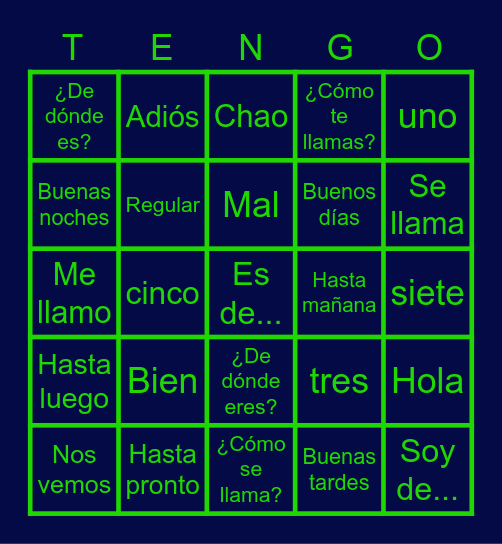The image depicts a Spanish-themed bingo card, consisting of a 5x5 grid of squares. The background is dark blue, while all elements, including the grid lines and text, are in neon green. At the top of the card, the letters "T-E-N-G-O" replace the traditional "B-I-N-G-O." Each of the 25 squares contains a different Spanish phrase or word, including greetings, questions, and common expressions. Notable entries include "¿De dónde es?" in the top left square, "adiós" in the second square, "ciao" in the third, "¿Cómo te llamas?" under the 'G' column, "uno" on the far right, "buenas noches," "regular," "mal," "buenos días," "me llamo," "hasta mañana," "bien," "tres," "hola," "nos vemos," "buenas tardes," "soy de...," and many more. The uniform neon green text on the dark blue background creates a striking visual contrast, clearly delineating each element of the card.